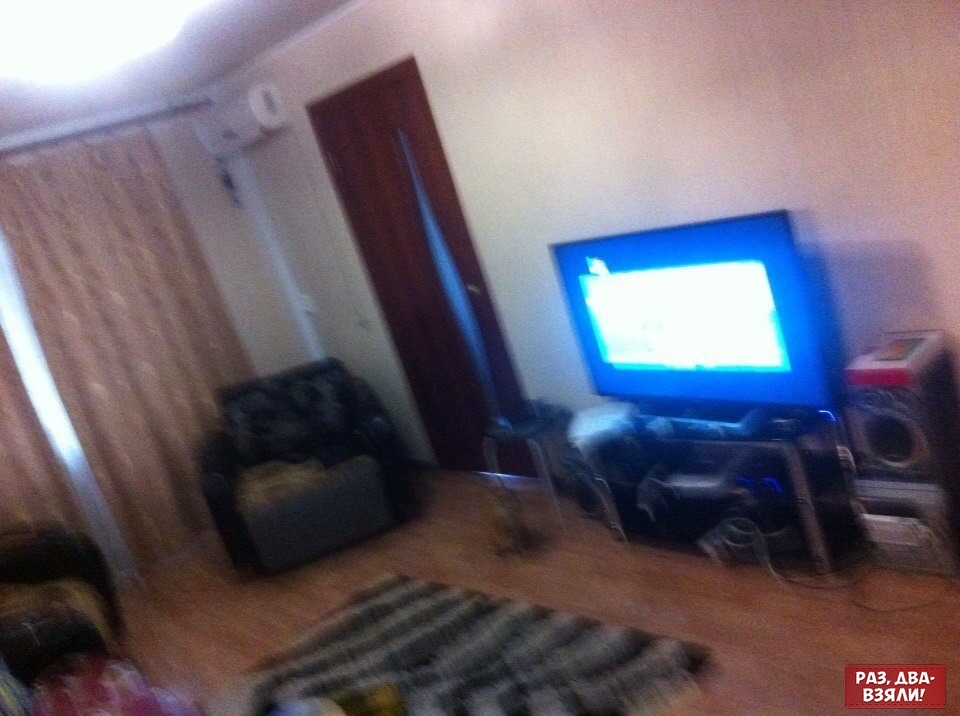The image shows a detailed view of a living room with various features. Central to the room is a small entertainment center consisting of a flat screen TV on a black and gray shelf. The TV is positioned against a white wall, which also has a large light fixture in the ceiling. Nearby, some electronics, possibly gaming devices, are situated under the TV. A speaker system is present next to the TV setup.

To the left of the entertainment center are two black recliner chairs. The floor features a light green and light gray striped rug, covering what appears to be a light wooden floor. The room also includes a dark brown door near the leather chair, and above this door, an air vent can be seen on the upper wall.

On the left side of the room is a large window adorned with full-length light brown curtains hanging from a pole fixed to the ceiling. Additionally, there is an open doorway with a red covering adjacent to this window. The image is slightly off-center, giving a slight tilt to the overall perspective.